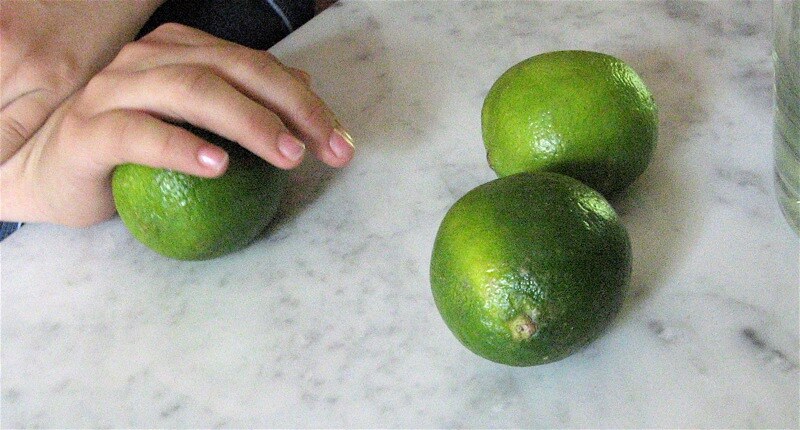In this detailed photo, three dark green, army-colored limes are displayed on a speckled marble countertop with gray and white patterns. Two limes are positioned towards the right-hand side, while the third lime is on the left, partially obscured by a person's hand. The person appears to be gently rolling the lime with their right hand, which has cut, unpainted nails and fair skin. The left hand rests on top of the right hand, making only a couple of knuckles visible. Additionally, a partially cut-off clear plastic bottle containing some liquid is seen to the right of the limes.